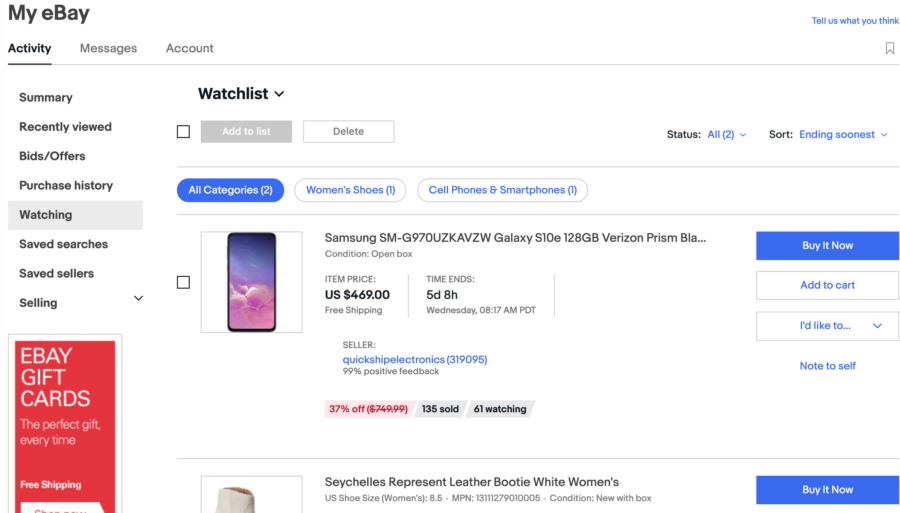The user is logged into their eBay account, specifically in the "My eBay" section. The interface displays three primary tabs at the top labeled: Activity, Messages, and Account. They are currently engaged in the "Activity" tab.

On the left side of the screen, there is a navigation pane featuring several options: Summary, Recently Viewed, Bids/Offers, Purchase History, Watching, Saved Searches, Saved Sellers, and Selling. The user has selected the "Watching" option.

The main section on the right now shows the user's Watch List. One of the items listed is a Samsung Galaxy S10e with 128GB of storage, compatible with Verizon, in black. The price is $469, and the auction is set to end in five days and eight hours. 

Another item visible, though partially obscured, is a pair of Seychelles Represent leather booties in white, intended for women. The items in the Watch List each have options to "Buy it Now" or "Add to Cart" next to their listings.